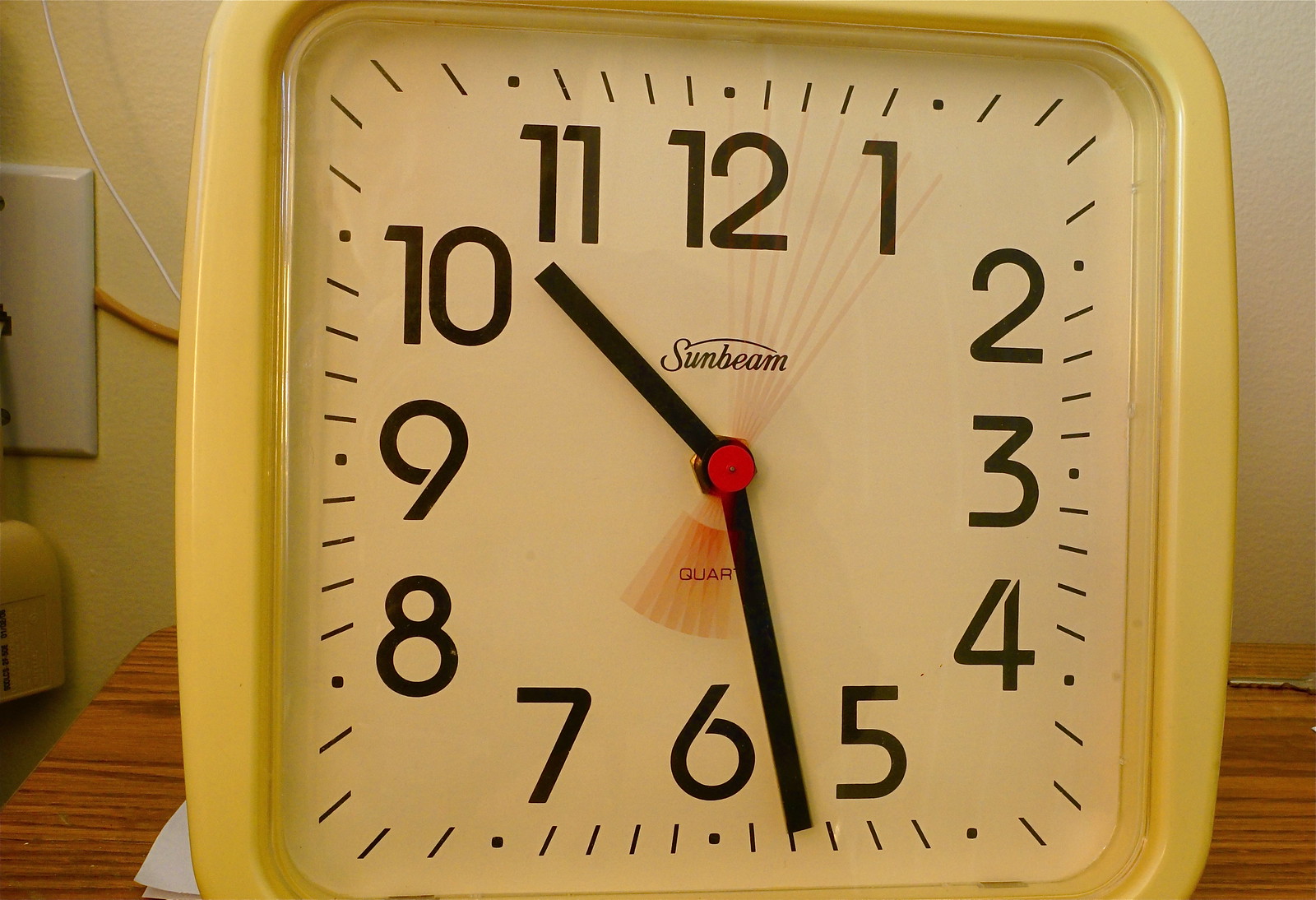This close-up photograph showcases a vintage square Sunbeam clock, likely from the 1980s, resting on a dark brown wooden table with visible wood grain and streaks. The clock, predominantly yellow with a creamy tint, features a white face detailed with black numbers and small black hash marks for precise time reading. The black hour and minute hands are accompanied by a red second hand, blurred between the 12 and 1, indicating motion. Central to the clock face, "Sunbeam" is elegantly inscribed in black cursive above a partially obscured "quartz" label, set against a subtle orange fan pattern. The surrounding environment includes a beige wall with a white outlet partially visible on the left, a yellow cord, and indistinct white objects behind the clock, adding to the nostalgic ambiance of the setting.